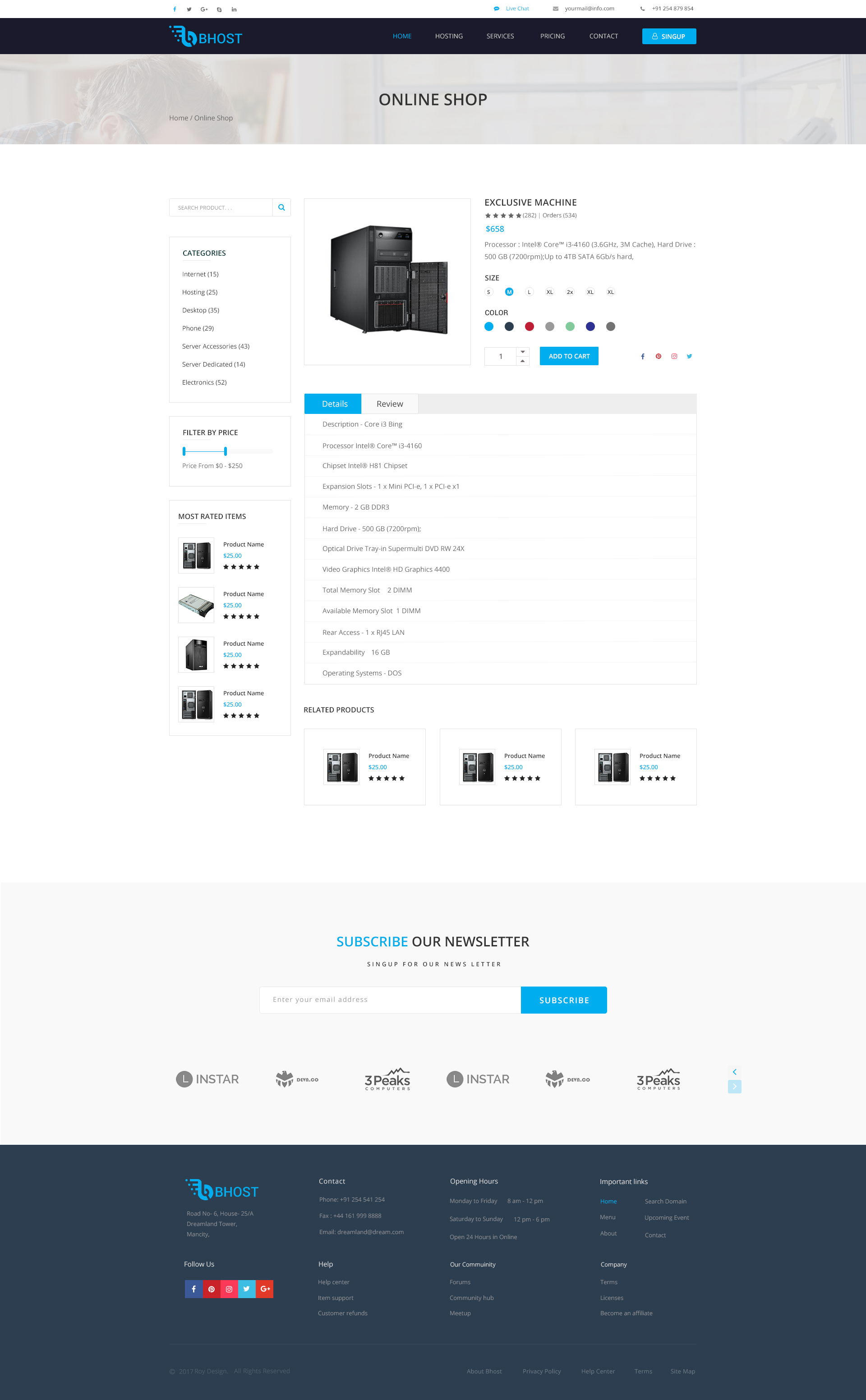The image depicts a desktop webpage from a site named "Behost" or something similar, featuring a prominent logo that is reminiscent of a hybrid between the Apple Beats and TikTok logos. Dominating the page is an image of a large server tower, labelled "Exclusive Machine," with a door swung open to reveal its internal components. Despite the text on the page being small and hard to read, the server tower noticeably stands out due to its substantial size and black color. The product appears to be highly rated with five-star reviews visible. Options for selecting different colors are present, along with an "add to cart" button. The size and appearance of the server tower make it seem unusually bulky, although this could potentially be a perception issue rather than the actual size of the device.